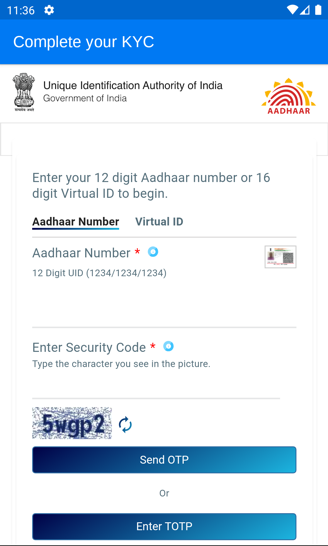**Detailed Caption for the Image:**

The image is a screenshot of a mobile application screen designed to facilitate the completion of the Know Your Customer (KYC) process. At the very top, a prominent blue banner displays the message "Complete Your KYC." Below this banner, the main content of the page is set against a white background.

On the upper section of the page, aligned to the left, is a distinctive logo. Adjacent to this logo on the right, in bold font, it reads "Unique Identification Authority of India." Directly beneath this in smaller, gray font, it states "Government of India." Accompanying this text on the right side is a colorful red and yellow sun-like icon or logo.

Moving down the page, a prompt instructs the user to "Enter your 12-digit Aadhaar number or 16-digit Virtual ID to begin," written in small gray letters. Below this instruction, there are two selectable options: "Aadhaar Number" and "Virtual ID," with the "Aadhaar Number" option currently selected, indicated by a small blue bar underneath it.

Following this section is a field labeled “12-digit UID” with an example shown in parentheses, where users are expected to input their Aadhaar number. Below this, in the left corner, there's a label that reads “Enter Security Code,” marked by a red asterisk indicating it is a required field. The text below instructs users to "Type the characters you see in the picture," referring to the CAPTCHA displayed beneath it.

At the bottom are two blue buttons: the first button, aligned to the left, is labeled "Send OTP," while the second one, aligned to the right, says "Enter TOTP." Centered between these two buttons is the word "or," offering users an alternative method to proceed.